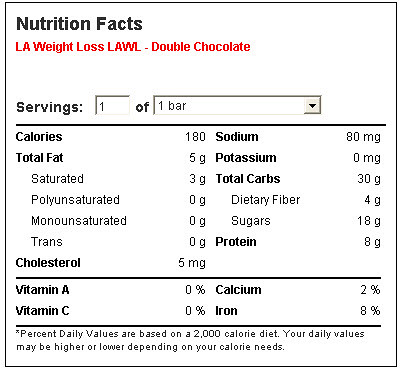This image displays the nutrition facts for an LA Weight-Loss (LAWL) Double Chocolate bar, which consists of two servings. Each individual serving provides 90 calories, totaling 180 calories for the entire bar. The sodium content per serving is 80 milligrams, with no potassium (0 milligrams) reported. The bar contains a total of 5 grams of fat per serving, of which 3 grams are saturated fat. It lists 0 grams of unsaturated or monounsaturated fats and 0 grams of trans fats. Notably, there is a discrepancy in the fat content as the remaining 2 grams are unaccounted for.